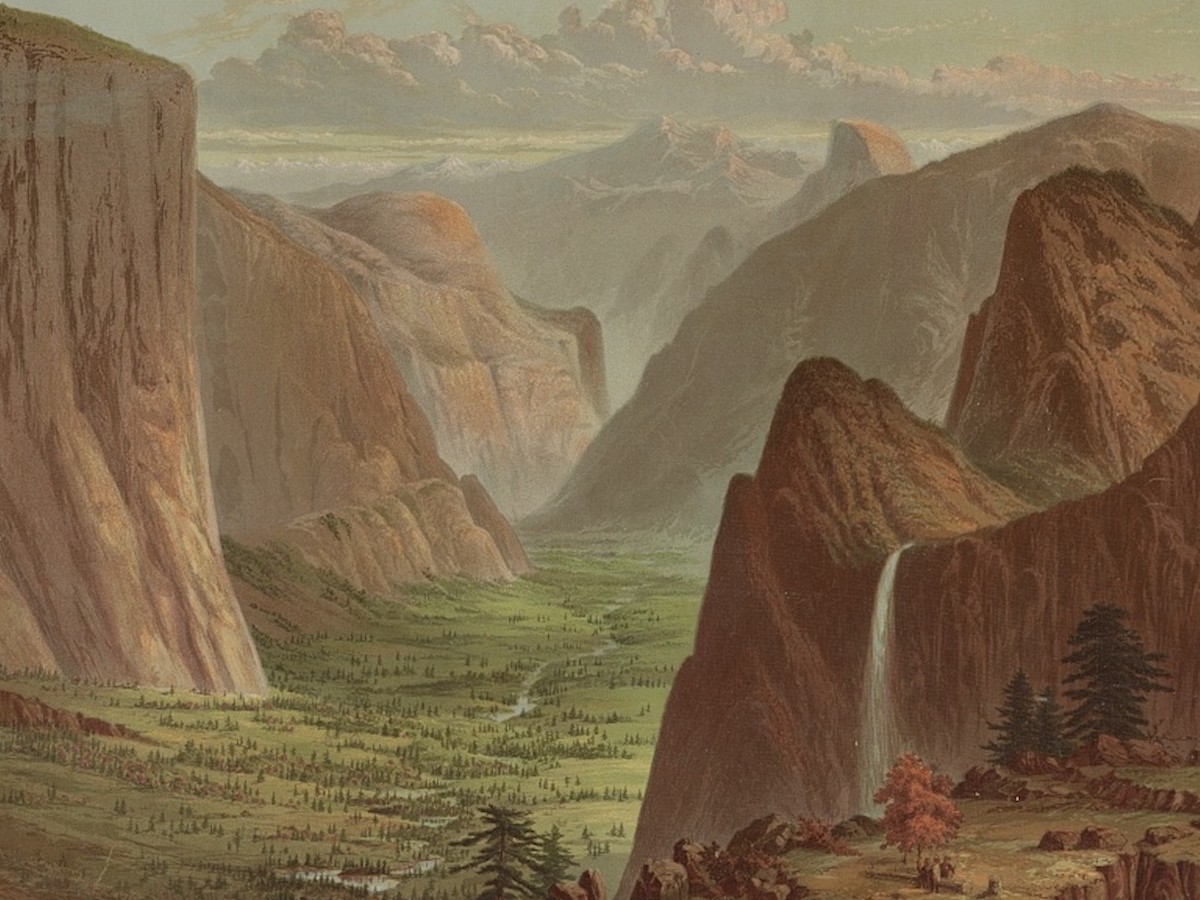This painting, likely an oil on canvas dating back 100-200 years, depicts a breathtaking canyon landscape. The scene captures the viewer's attention with its sprawling vistas and detailed elements. At the heart of the composition lies a lush, green valley adorned with grass, trees, and a slender, meandering river that flows from the foreground to the distant horizon. Flanking the valley are towering red rocky formations and desert-like clay mountains, creating a dramatic contrast against the vibrant greenery. To the right, a prominent rocky cliff features a delicate waterfall cascading down, though its destination is obscured by another rock formation. The sky above is richly painted in shades of light green, blue, and gray, filled with textured clouds. The sense of depth and natural beauty is further enhanced by additional mountain ranges fading into the distance, making this picture truly captivating.